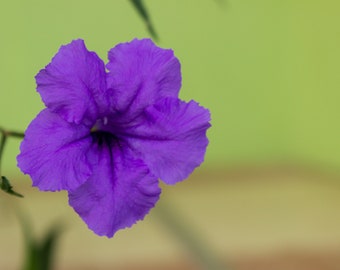The photograph is a detailed close-up of a vibrant purple flower, likely a morning glory, taken in portrait mode. The flower, occupying most of the foreground, has five distinct petals with no visible pollen in the center, displaying a rich, vibrant hue. Behind the flower, a thin green stem emerges but becomes blurred into the background. The background itself is predominantly green, occupying the top two-thirds of the image, transitioning to a tan hue in the bottom portion. Despite being out of focus, you can make out the fuzzy outline of a darker green branch and a few leaves, which likely belong to the same flower's plant. Notably, there is a triangular blade of dark green grass descending from the top and another small, blurry leaf near the middle, adding to the scene's depth and texture. Overall, the blurred green and tan backdrop highlights the delicate purple bloom as the focal point of this simple yet striking photograph.